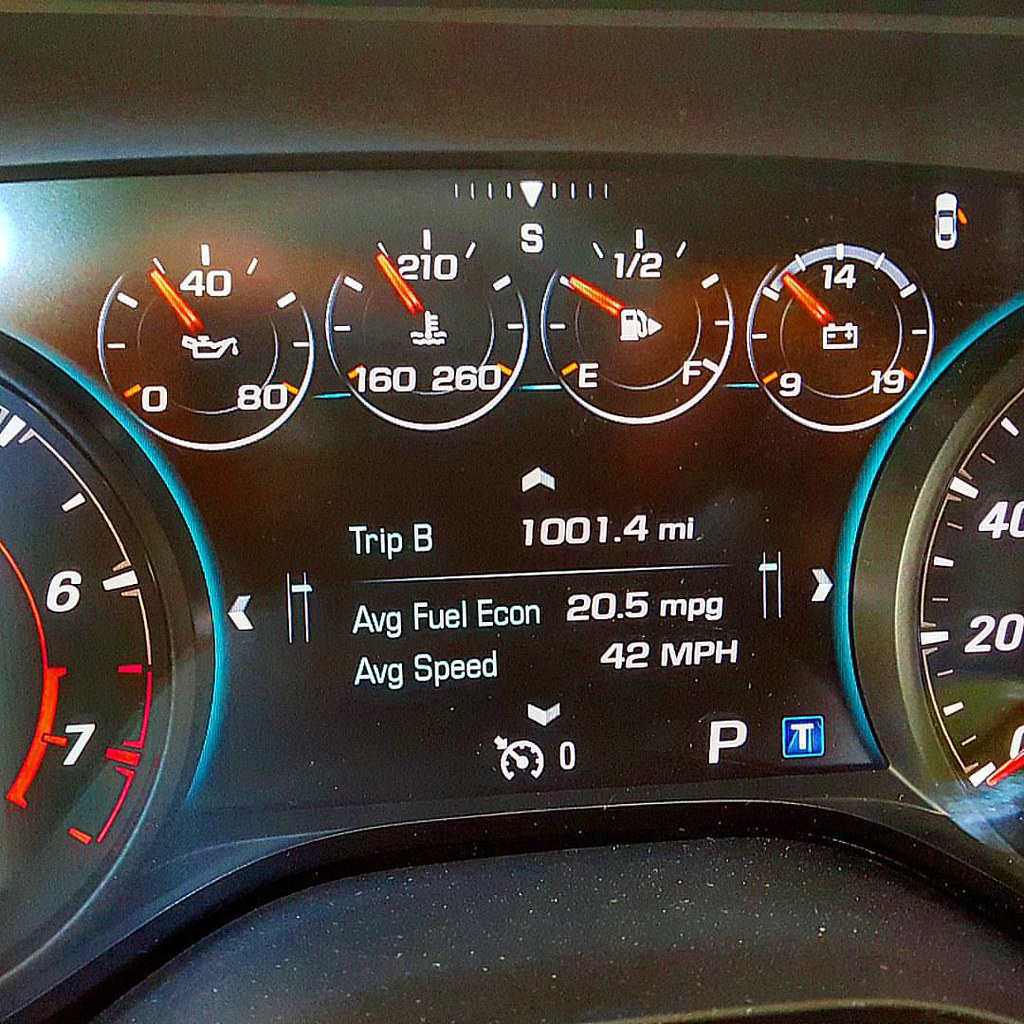This image depicts a close-up view of a car's black dashboard, featuring four circular gauges with detailed markings. Two large circles on either side house red dials and red and white indicators, showing various metrics such as fuel levels, oil temperature, and battery power. Within these circles, detailed digital readouts provide information, including "Trip B: 1001.4 miles," "Average Fuel Economy: 20.5 miles per gallon," and "Average Speed: 42 miles per hour." Additional indicators show a small gauge with a needle pointing to zero, a "P" symbol, and a blue "T." The background is mostly black, with all letters and numbers displayed in white, enhancing readability and allowing for easy monitoring of vehicular statistics. The sophistication of this dashboard technology helps the driver manage and plan future trips efficiently.